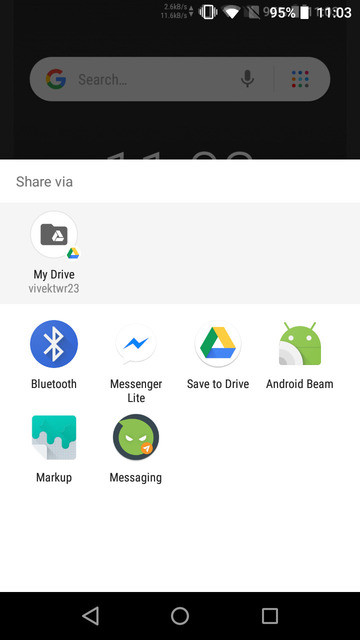This image is a detailed screenshot from a smartphone. At the top of the screenshot, the header is black with white text. In the upper right-hand corner, the time displayed is either 1:03 or 11:03, accompanied by a battery icon showing a 95% charge. Next to the battery icon is the Wi-Fi icon, depicted as an inverted triangle, and an icon indicating that the phone is on mute.

Below the header, the screenshot shows the Google Search engine homepage. The search box appears in a very dark gray shade, while the Google logo is also somewhat dark, likely due to the overall darker background.

Continuing downward, the background turns white. In the upper left-hand corner of this white section, the text 'Share via' is displayed in a fine gray font. Below this, 'My Drive' is mentioned with its icon—a gray folder featuring a small white triangle.

In the next row, running from left to right, are several icons: Bluetooth, Messenger, Light, Save to Drive, and Android Beam. Below these icons are options for 'Markup' and 'Messaging'. The bottom border of the screenshot is in the same black color as the header.